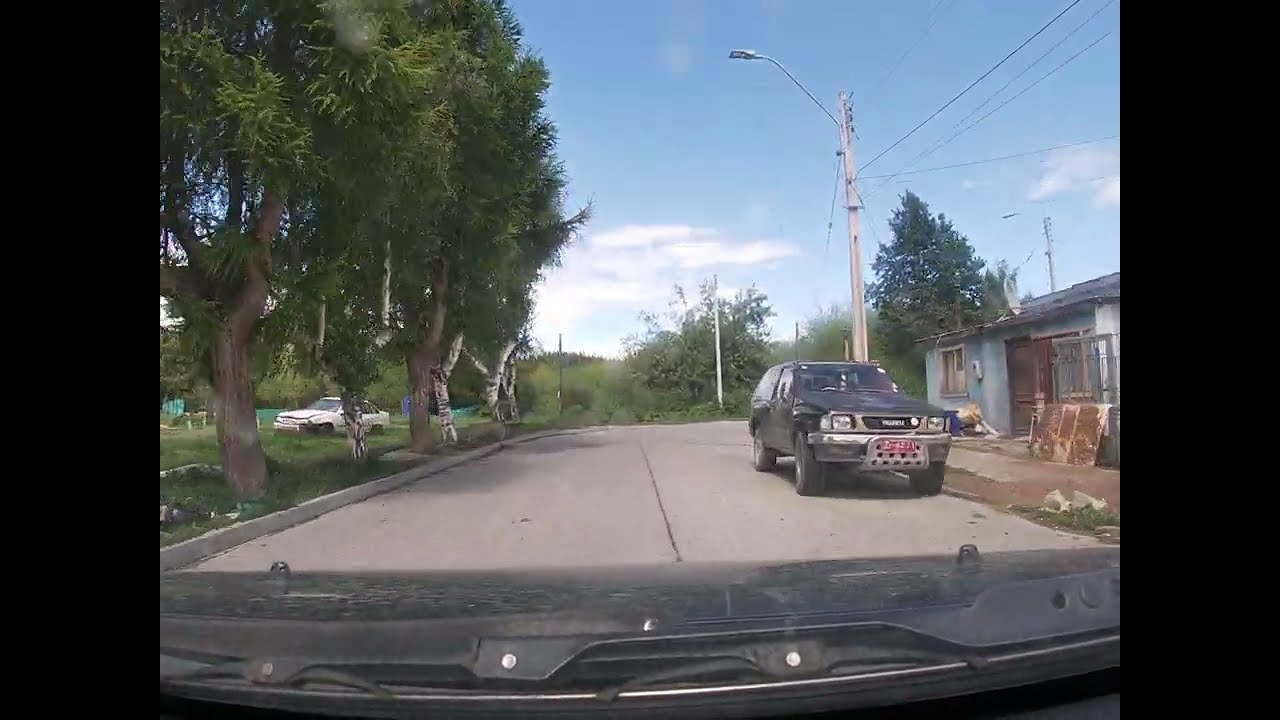The image appears to be taken from inside a vehicle, with part of the car's windshield visible at the bottom. Through the windshield, a small, somewhat old asphalt street can be seen, bordered by various elements. On the right side of the road, a dilapidated light blue house with a flat roof stands, looking worn and surrounded by debris. Next to this house, a black truck with a black hood is parked. Adjacent to the truck is a dirt patch, followed by a streetlight and electrical wires crossing above in the sky. The left side of the street boasts tall grass and an array of trees, including two large brown trees and several thinner ones with lush green leaves. Amongst the trees, a white car is parked on the grassy area, possibly broken down. The scene is set against a clear, blue sky dotted with a few sparse, wispy white clouds.